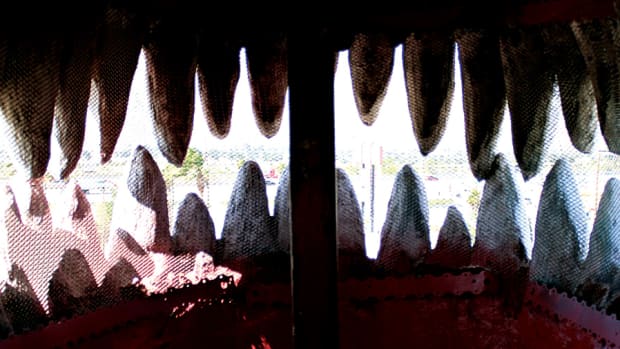The photograph is a captivating view from inside what appears to be a large sculpture of a carnivorous creature's mouth, possibly an exhibit at an amusement park or museum. The perspective offered places the viewer as if they were inside the mouth of a gigantic reptile or dinosaur, with sunlight streaming in through the open jaws. The interior of the mouth is predominantly red, and the teeth are long, cylindrical, and plantain-like in shape, tapering down to rounded points. These teeth are fairly separated and organized in groups of five or six, all supported by visible metal braces and a large metal bar in front. Observers from inside can see a partially-obstructed view of the outside, including a bright sunny day, glimpses of trees, and some grass, though the broader details of the scene outside are unclear due to resolution and shadowy lighting from within the sculpture. Some teeth even appear to touch each other, adding to the intricate structure of this fascinating installation.